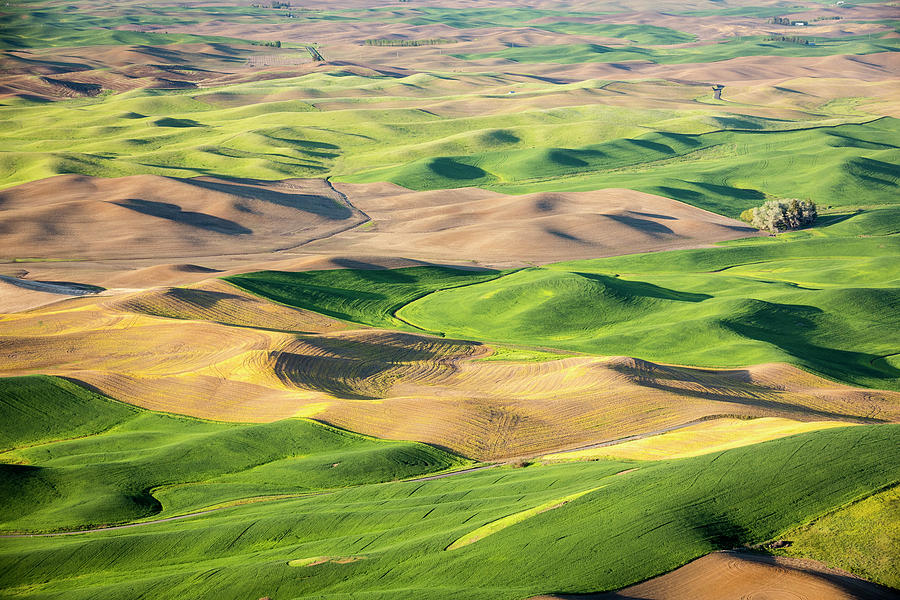The image appears to depict an artistically rendered aerial view of a rural landscape with rolling hills and a patchwork of fields. The land is divided into sections with flowing shades of green, yellow, brown, and other earth tones, indicating areas of grass, dirt, and crops. The terrain is uneven and mildly hilly, with various colors blending together to create a richly textured scene. Notably, the image lacks any people, animals, or buildings, creating an expansive, untouched feel. 

In the bottom right corner, there is a noticeable diagonal patch of lemon-yellow color, which could represent a pile of gathered crops or a distinct section of land. Small trees or shrubs are scattered sporadically throughout the landscape. The view is from above, suggesting it could be an aerial or drone photograph, though the image also carries stylistic elements that resemble a painting or a photograph with special effects filters. The area appears to be deserted under daylight, and the presence of shadows adds depth and contrast to the scene.